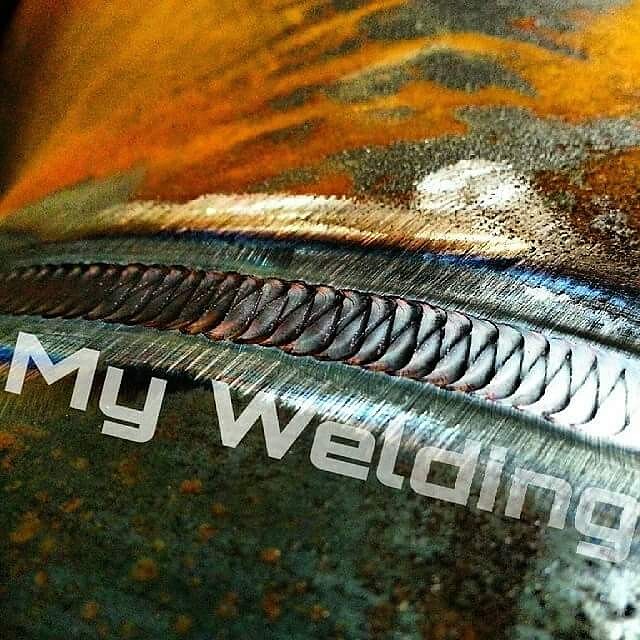This is a highly detailed, close-up square image featuring a metallic zipper chain prominently running from the center left to the bottom right, creating a curved line. The zipper chain is silver in color with accents of green and brown, hinting at some wear or possible use. Surrounding the zipper on its right side is a fabric that varies in shades of yellow with shiny undertones, while on the left side, the fabric transitions into green with yellow spots, interspersed with brown and orange accents. The overall color scheme includes hints of rust and darker green, giving it a textured and multi-hued appearance. The photograph is taken straight on, emphasizing the fine details of the zipper and the fabric. A watermark reading "My Welding" in large, transparent white font is distinctly visible at a diagonal from the bottom left to the top right. The setting suggests that the image was likely taken inside a shop or on a work table, focusing strictly on the zipper and the fabric's texture.